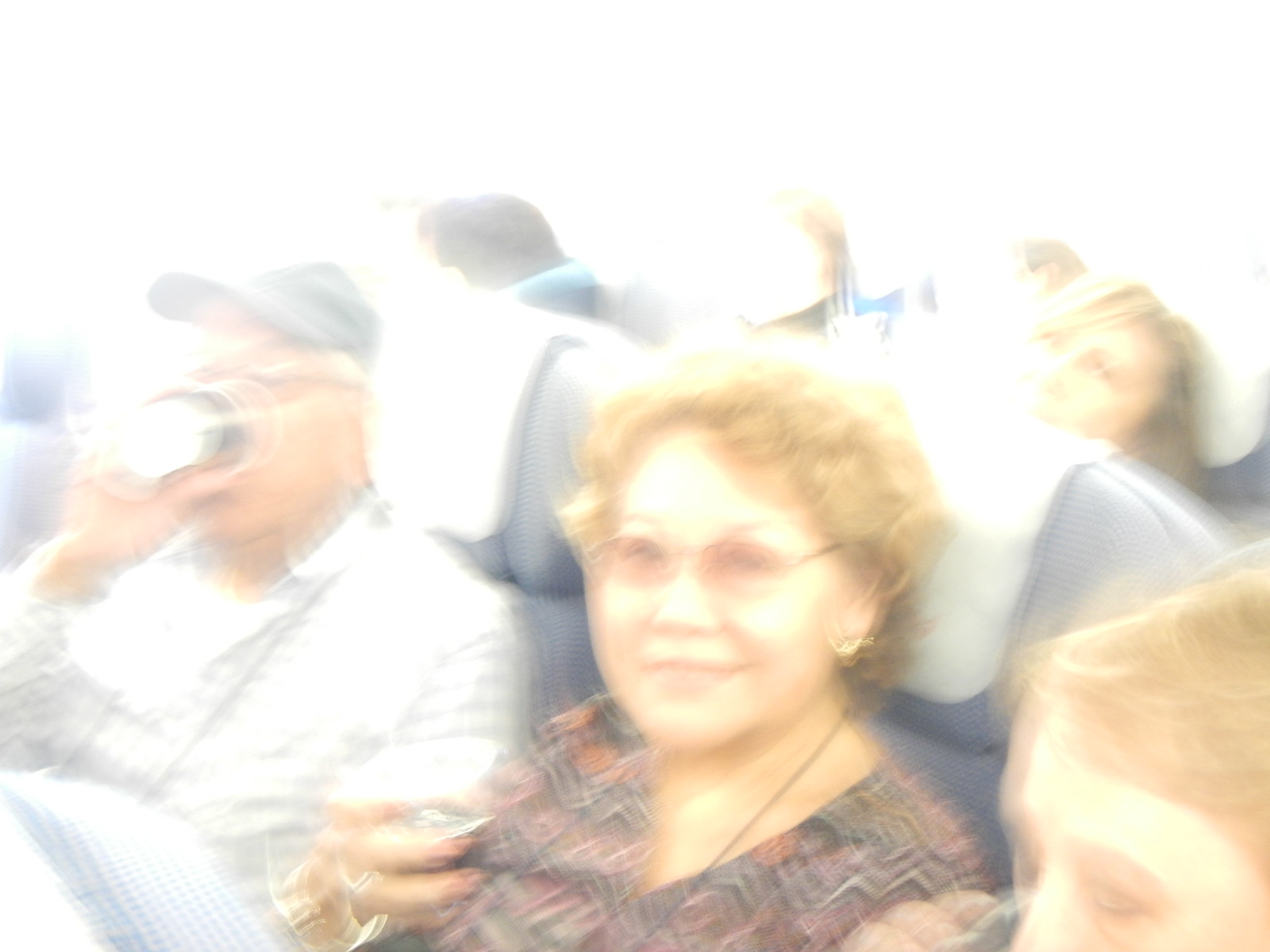This photograph captures a group of individuals seated closely together inside an airplane, with seats aligned in rows of three across. The airplane seats are blue with dotted patterns and feature gray-colored headrests. The entire image is overexposed, resulting in a bright, washed-out appearance, especially noticeable in the areas to the left and above the individuals in the front, as well as a generally grainy texture.

In the foreground, a woman with short, reddish-blonde hair and sunglasses wears a black, red, and pink zigzag striped top. She holds a glass in her right hand and is seated next to a man in a white shirt and gray baseball cap, who is drinking from a cup. To her immediate right sits another woman with blonde hair, and in the row directly behind, another blonde-haired woman can be seen looking towards the camera. Additionally, a man wearing a black hat and a white and black striped shirt is visible, also sipping from a drink. The image, although not very clear, depicts a lively and cramped setting typical of a commercial airplane flight.